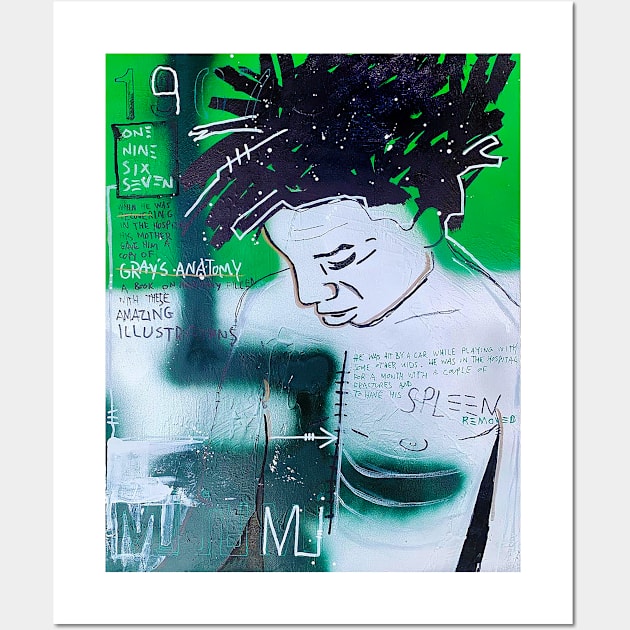This is an illustrative poster with a light gray background and a white border, featuring a Basquiat-style image. At the center is an African-American man depicted with light gray painted skin and short black dreads, drawn in a collage-like fashion with black rectangles. He is looking down at his chest, which appears to be cut open, showing a detailed scar that indicates his spleen has been removed. The backdrop of the heads is prominently lime green.

In the top left corner, the numbers "1967" are displayed in varying shades of green and white, with additional text stacked underneath outlining the background story: the man was hit by a car while playing and spent a month in the hospital with multiple fractures and undergoing spleen removal surgery. His mother gave him a copy of Gray's Anatomy during his hospital stay, a detail noted in the poster. Various handwritten elements and titles, including "Gray's Anatomy," are scattered across the print, adding to its collage-like aesthetic. The lower portion of the poster features blue and light blue tones, contrasting with the green upper section.